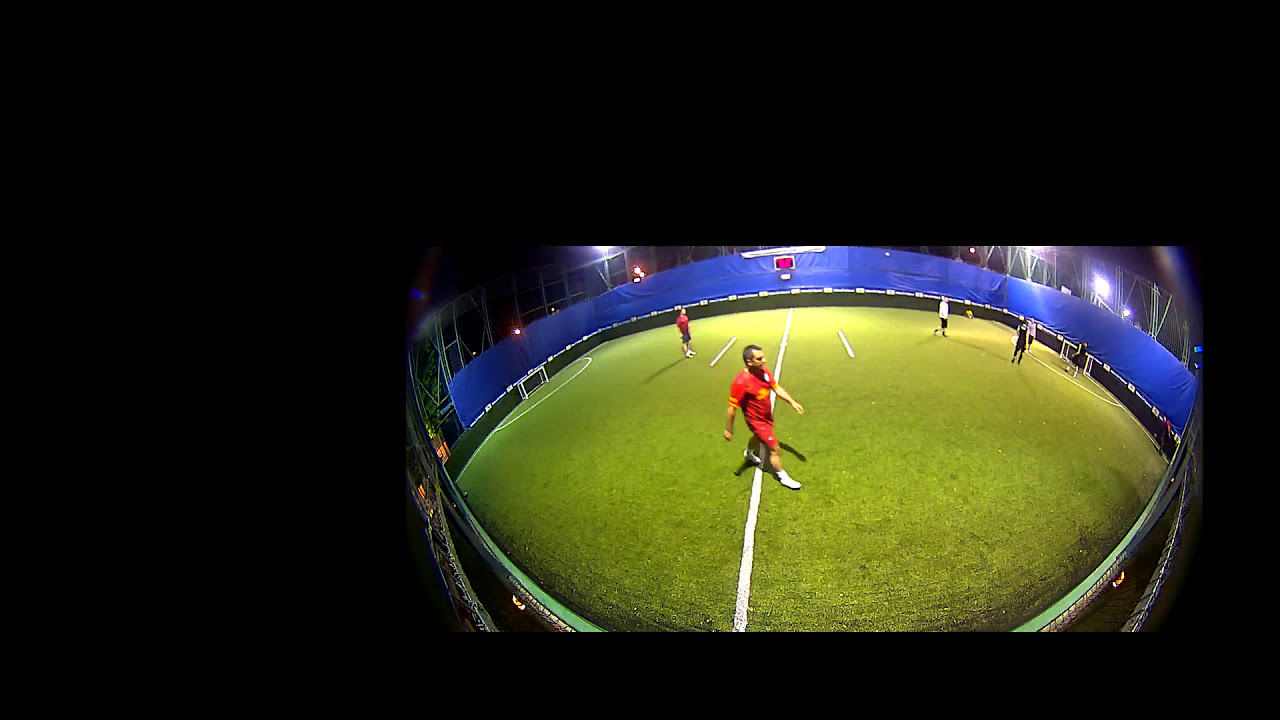The image captures a night scene on a neatly groomed outdoor soccer field surrounded by a blue fence-like border. Visible under the illumination of white, red, and green lights, the grassy field is marked with white chalk lines that likely separate the teams. A few men in red uniforms with white sneakers are seen prominently in the center, while others in black and white uniforms, possibly referees, add to the mix. The setting includes the upper part of the dark sky and stadium lights, hinting at a game that might have recently concluded, given the sparse presence of players. The empty surrounding areas accentuate the focus on the field, contributing to the overall serene yet anticipative atmosphere of the scene. No text is visible in the image, but the colors stand out against the night backdrop, including hints of blue, green, white, red, yellow, and orange.